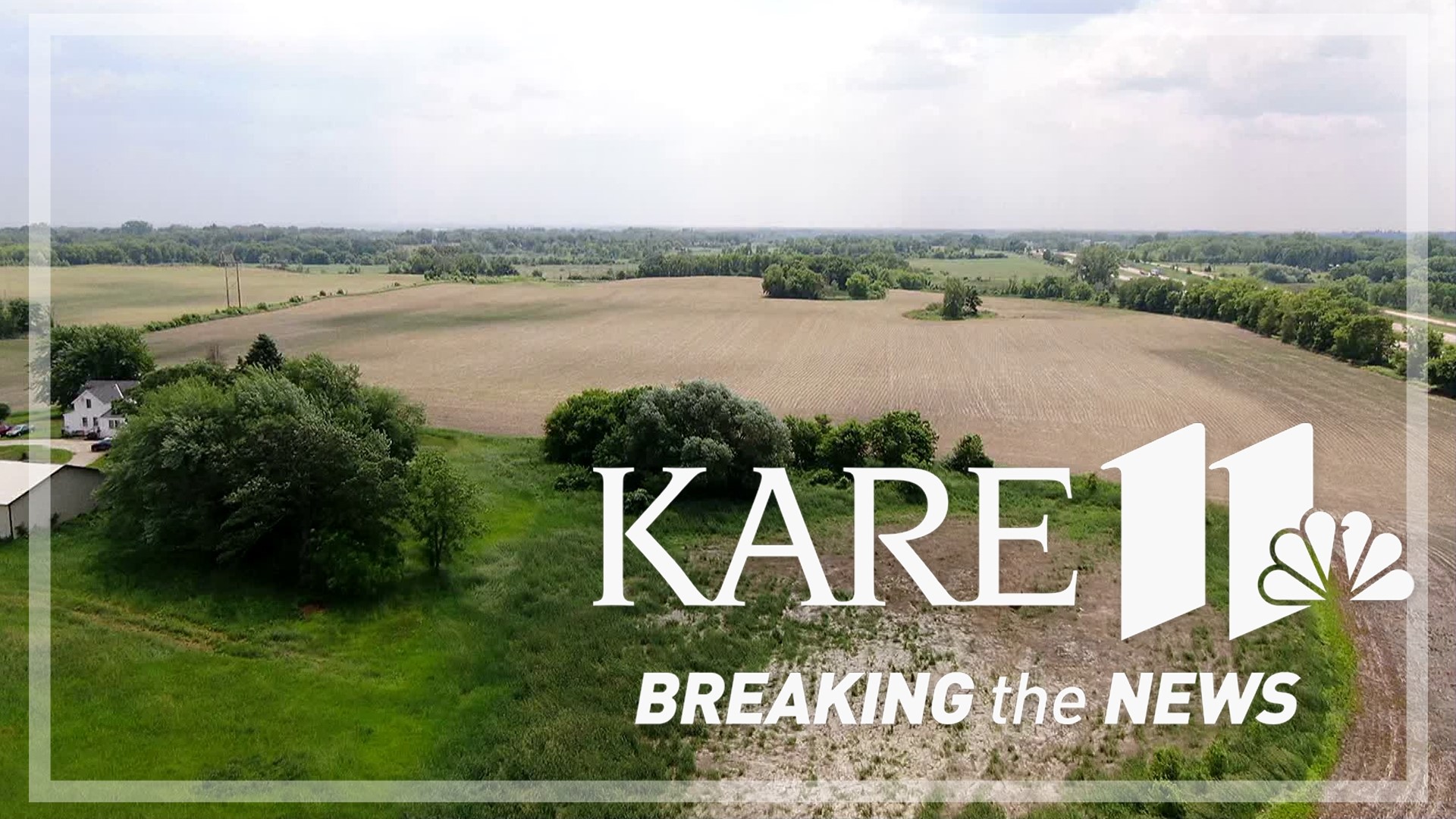The image depicts a vast farmland on an overcast day, viewed from an elevated perspective, possibly from a low-flying plane. The field, recently cultivated and currently barren, is surrounded by a mix of trees. On the horizon, more trees can be seen under the cloudy sky. In the left-center of the image, there is a white farmhouse with some cars parked outside and a white warehouse-like building nearby. Off in the distance, on the upper right side, cars are visible traveling down a highway. Overlaid on the image, in bold white letters, are the words "KARE 11" followed by the NBC Peacock symbol and the phrase "BREAKING THE NEWS." The photograph serves as both a visual of the tranquil rural landscape and an advertisement for the KARE 11 news channel.